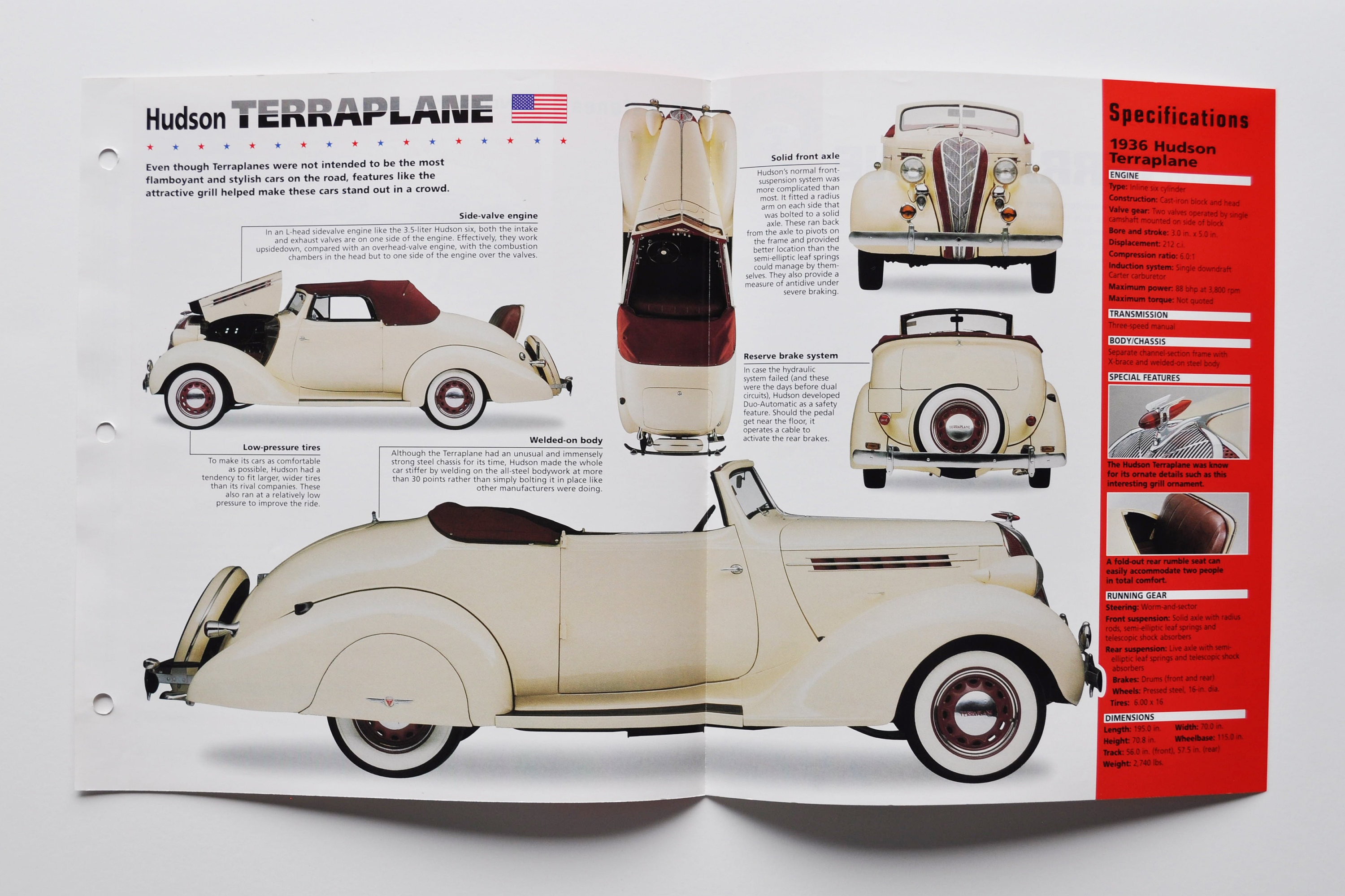This detailed image depicts a two-page magazine spread from a vintage publication, showcasing the 1936 Hudson Terraplane automobile. The spread features five distinctive views of the car: from the top, the front, the back, and each side, highlighting its cream-colored body with a retractable dark brown convertible top. The Terraplane is displayed with notable elements like its spare wheel and cover at the rear, the latter featuring a white outer edge and a brown center. The front of the car is adorned with a prominent chrome grille flanked by two chrome headlights, and a slim chrome bumper extending across the front. In the upper left corner, the text "Hudson Terraplane" is accompanied by an American flag, underscoring its heritage. To the right, against a red backdrop, there is detailed text listing the specifications of the car, including the engine, transmission, body details, special features, dimensions, and running gear. This advertisement emphasizes the car's practical yet stylish design, particularly noting its attractive grille as a standout feature.